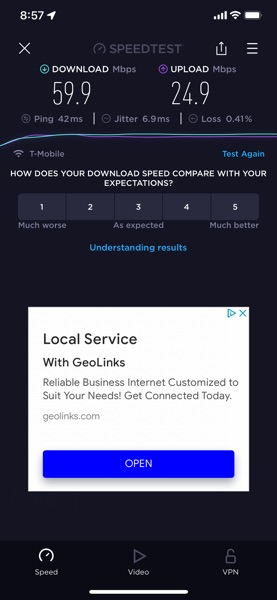The image features a smartphone screen displaying the results of a speed test conducted on the T-Mobile network. At the top left corner, the screen shows the time as 8:57, along with four signal bars, a full Wi-Fi signal, and a fully charged battery indicator. Just below this information, there's a small 'X' icon on the left.

In the center of the screen, the app's interface features a speed test result with the heading "Speedtest" accompanied by the Ford symbol and three horizontal lines stacked on top of each other. Directly beneath this header, the download speed is displayed as "59.9 Mbps" and the upload speed as "24.9 Mbps." 

The next section down provides more detailed metrics: to the left, the ping is noted as "42 ms," followed by jitter at "6.9 ms," and packet loss at "0.41%." 

Below these metrics, the text "T-Mobile" appears. Adjacent to it, a blue hyperlink labeled "Test Again" offers the option to rerun the speed test.

Further down the screen, a prompt in white, capitalized letters asks, "HOW DOES YOUR DOWNLOAD SPEED COMPARE WITH YOUR EXPECTATIONS?" Beneath this question, there are five boxes numbered one through five, with the text "Much Worse" on the far left and "Much Better" on the far right, and "As Expected" positioned centrally.

The image description concludes with a blue hyperlink at the bottom that reads "Understand the Results."